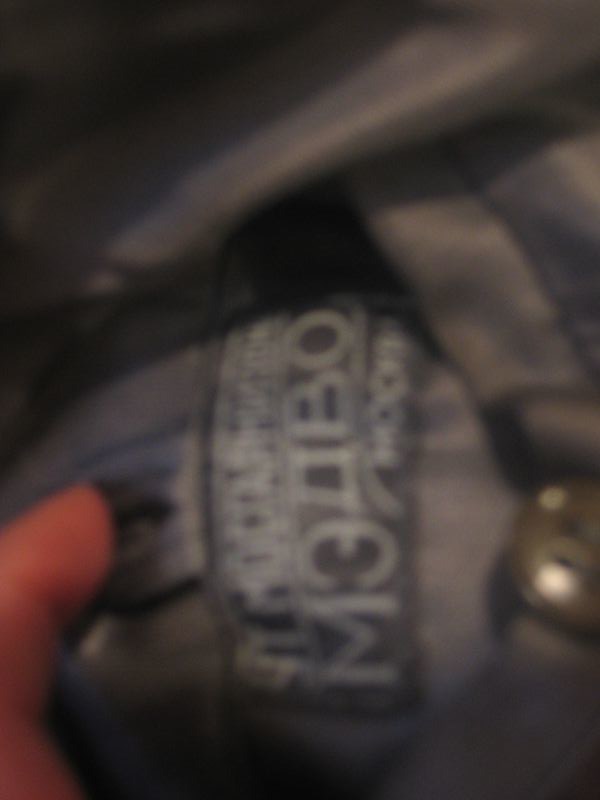The image is a very blurred and poorly lit photograph, adding to the challenge of discerning its contents. On the left side, a human finger, focused mainly on the fingertip up to the middle knuckle, appears to be pressing down on something. This object may be a black or dark grey piece of fabric, possibly faux leather or denim, displaying a label or patch with white text, oriented vertically and very difficult to decipher. The fabric exhibits wrinkles and a reflective quality. On the right, a small metal button is visible, suggesting a piece of clothing or accessory. The unclear context and the angle from which the photo is taken add to the overall ambiguity of the image's details.